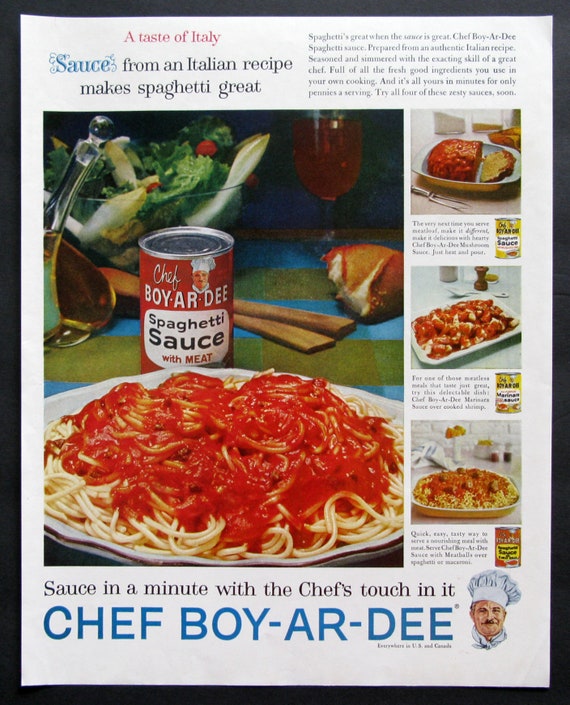This vertically aligned rectangular magazine advertisement features a thin, quarter-inch black border around a white background. At the very top left corner, in red text, it reads "A Taste of Italy," followed by a blue heading, "Sauce from an Italian Recipe Makes Spaghetti Great." Immediately to the right of this headline is a justified paragraph in black text discussing the delights of spaghetti.

Dominating the left side of the page is a large, indoor photograph showcasing a white plate brimming with spaghetti drenched in rich tomato sauce. Positioned just behind the plate is a vividly colored can of Chef Boyardee Spaghetti Sauce with Meat, complete with a vibrant red label and an illustration of a chef in a large French hat. A bowl of salad is subtly visible in the distant background. 

To the right of this main image, arranged vertically, are three smaller images, each accompanied by a brief descriptor underneath. These images depict different culinary creations made with Chef Boyardee sauces – the top image resembles a meatloaf, the middle seems to be a seafood shrimp dish, and the bottom features spiral noodles topped with meatballs.

At the bottom of the page, the text boldly states, "Sauce in a Minute with the Chef's Touch in it." Directly below this in large, blue all-caps letters is "CHEF BOYARDEE," accompanied by an illustration of the iconic chef's head in the bottom-right corner.